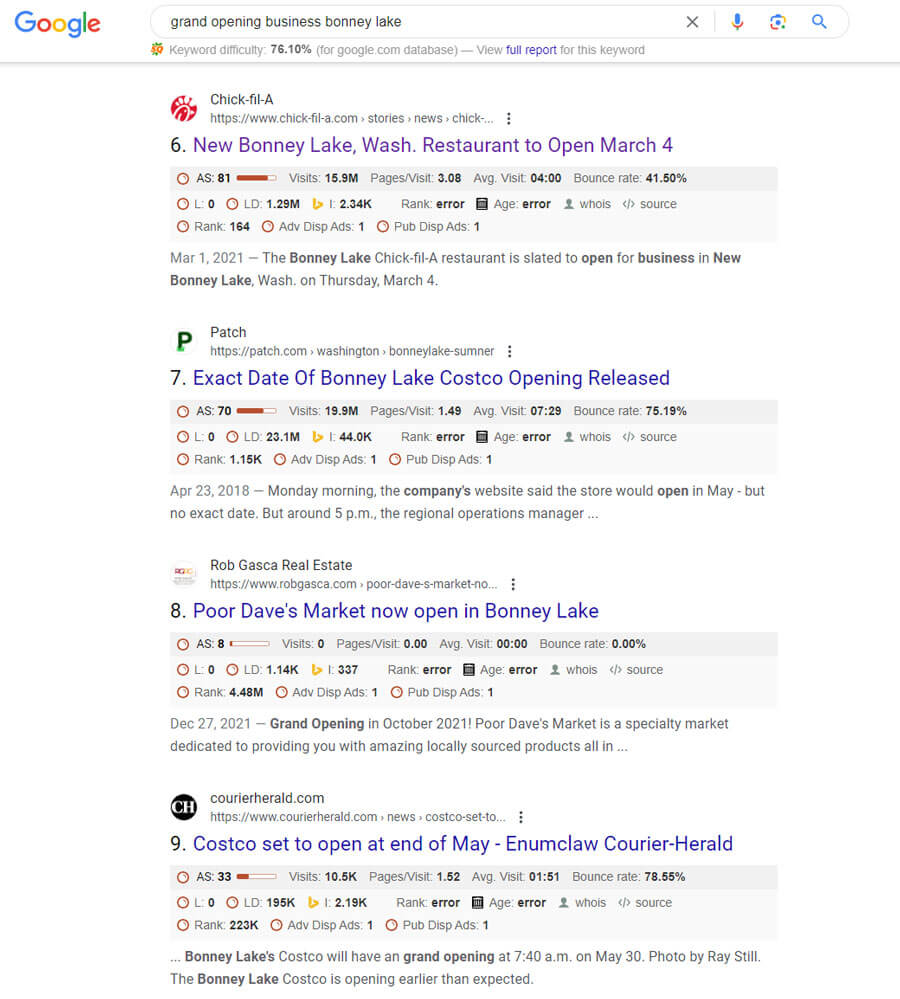This is a detailed screenshot taken of a section of a Google search results page, captured in a portrait orientation. At the top left corner of the screenshot, the iconic Google logo is displayed in its recognizable sequence of blue, red, yellow, blue, green, and red letters. Next to the logo is the search box, containing the search query in black text. Adjacent to the search box on the right, there is an X icon for clearing the search, followed by three multicolored icons: a microphone for voice search, a camera for image search, and a magnifying glass for executing the search.

Below this header, the background transitions into plain white, showcasing four different search result links related to the query.

1. The first result is for Chick-fil-A. The entry begins with a red circle featuring a white cartoon chicken head. To the right, "Chick-fil-A" is written in black text, with the website address below also in black. Beneath this, in purple text, there are statistical details about the restaurant and its website, including metrics like visits, pages per visit, average visit duration, and bounce rate, each accompanied by relevant icons.

2. The second result starts with a green "P" icon on the left corner. To the right, the word "PATCH" appears in black text, with the website address immediately below in a smaller font. The entry mirrors the structure of the first result, providing similar webpage statistics, followed by a brief content description in black text.

3. The third result features a white circle with red text and a logo. To the right, the website name is displayed in black text. Below, in larger blue text, the website address is shown, followed by the familiar set of website statistics from the previous results. A short introductory sentence in black follows.

4. The final result presents a black circle with the letters "CH" in white as its icon. To the right, the website name is indicated in black text, accompanied by the website address below in smaller black text. The address is followed by larger blue text that denotes the webpage title. This result also includes the standard three-line statistics, concluded by a two-line preview of the web page's content in black text.

Each search result is clearly delineated, ensuring a user-friendly interface and easy navigation through the provided information.